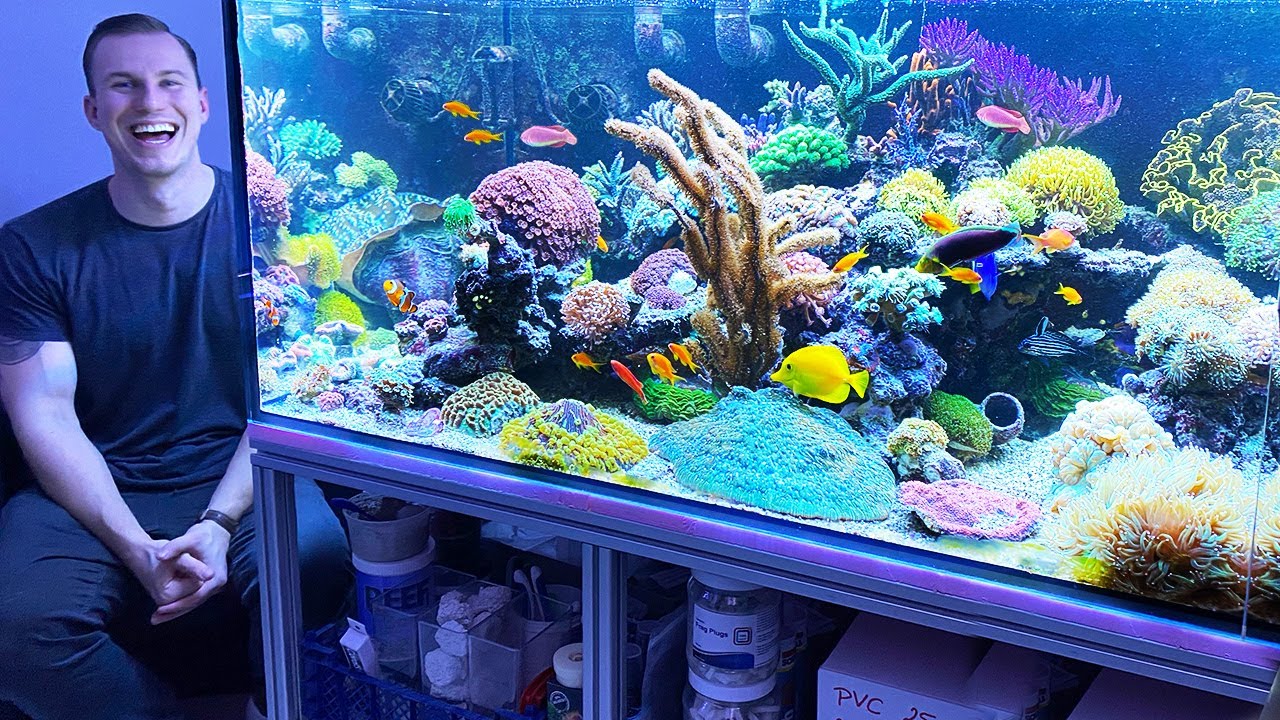This image features a man sitting on the left-hand side next to a large, vibrant home aquarium. The man, who has short brown hair, is wearing a black t-shirt that partially reveals a tattoo underneath, along with a watch and dark jeans. He is smiling widely, almost laughing, with his hands clasped together between his knees, showcasing his affable demeanor. The aquarium is quite substantial, roughly two feet tall and five feet wide, and is densely populated with a variety of tropical fish and aquatic plants. The fish tank contains yellow fish, blue fish, orange fish, a clownfish, and a larger yellow fish with a distinctive snout. The tank is filled with colorful decorations including coral, rocks, and various forms of seaweed and seagrass, leaving virtually no empty space. Below the aquarium, there are storage compartments holding fish food, maintenance supplies, plastic boxes, and clear containers filled with items like cotton balls and Q-tips, essential for keeping the aquarium in pristine condition. The man’s joyful expression and the lush, lively aquarium create a vibrant and engaging scene.